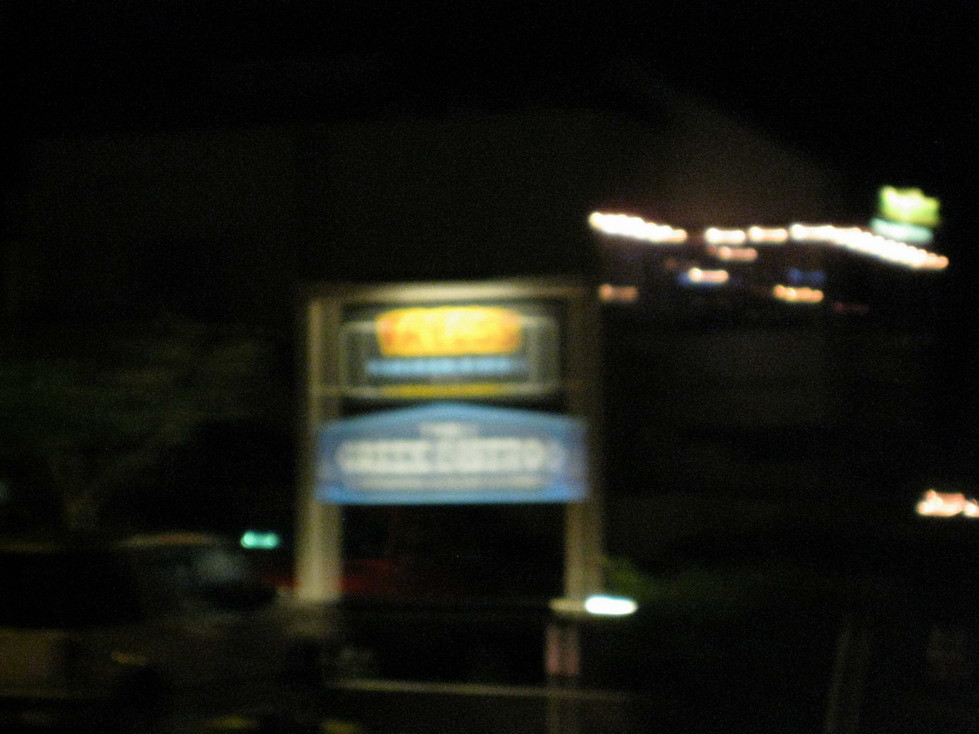The photograph captures a nighttime scene enveloped in darkness, devoid of visible skies or stars. In the foreground, a blurred signpost adorned with blue and white signs stands prominently, slightly illuminated by a yellow light at its top. To the left of the signpost, the indistinct outlines of one or two vehicles can be discerned. On the right side and further in the background, a brightly lit building punctuates the darkness, adding a contrasting light source to the otherwise pitch-black scene.